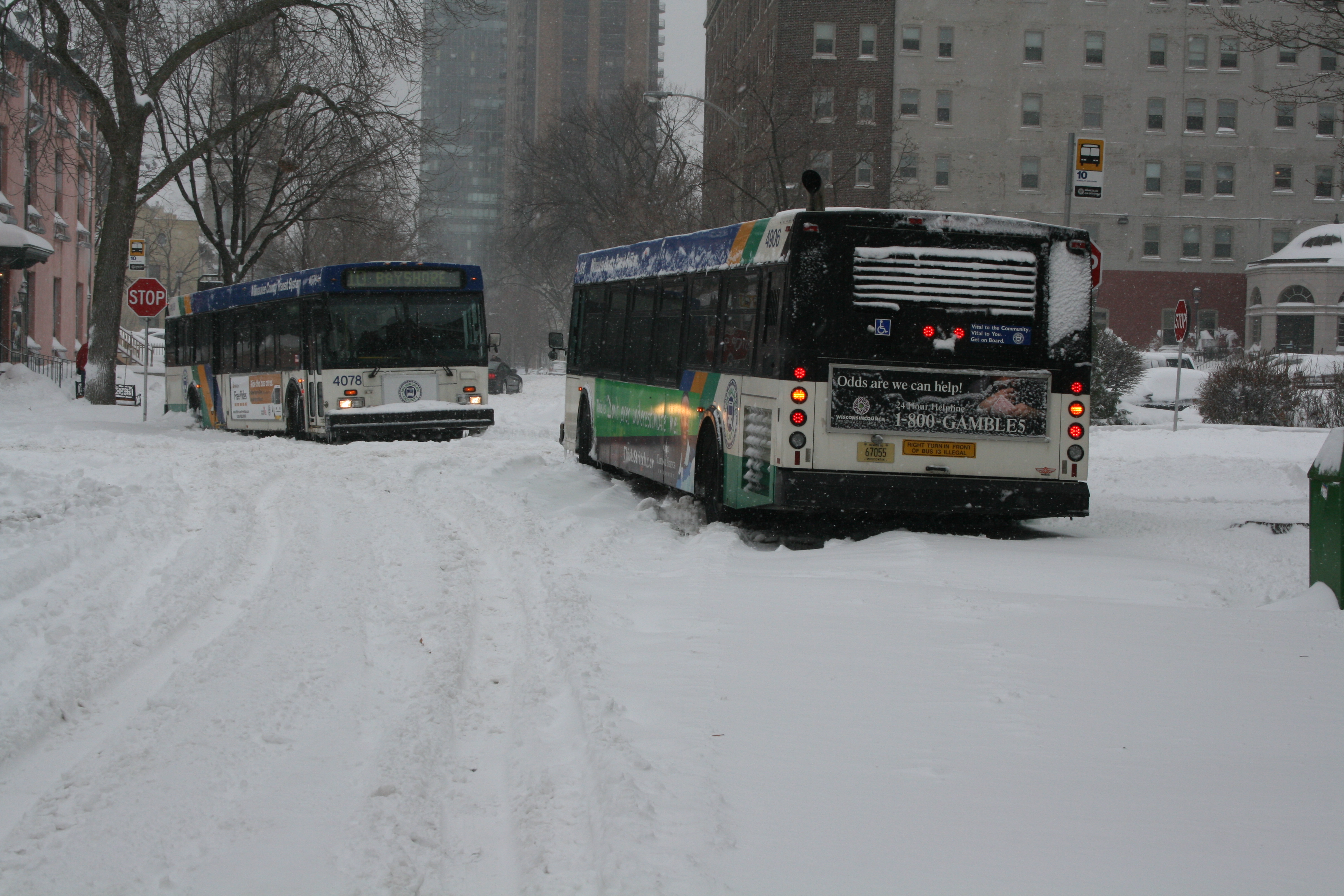In the midst of a heavy snowstorm in a bustling urban landscape, two city buses navigate a snow-covered street. One bus heads away from the camera while the other approaches, creating a dynamic sense of movement despite the challenging conditions. The deep, unplowed snow has left prominent tracks on the road, suggesting the buses may be struggling to proceed. Both buses are primarily white, adorned with green, yellow, blue, and orange stripes, and have their headlights and various lights turned on. The more prominent bus in the foreground features an advertisement with the text "odds are we can help 1-800-gambles, gamble 5." Surrounding the street, one can see a red stop sign, trees, and a blue mailbox, all partially buried in snow. Encircling the scene are various buildings, including large apartment complexes and possibly a high-rise office or residential building in the distance, completing a vivid picture of urban life grappling with harsh winter weather.